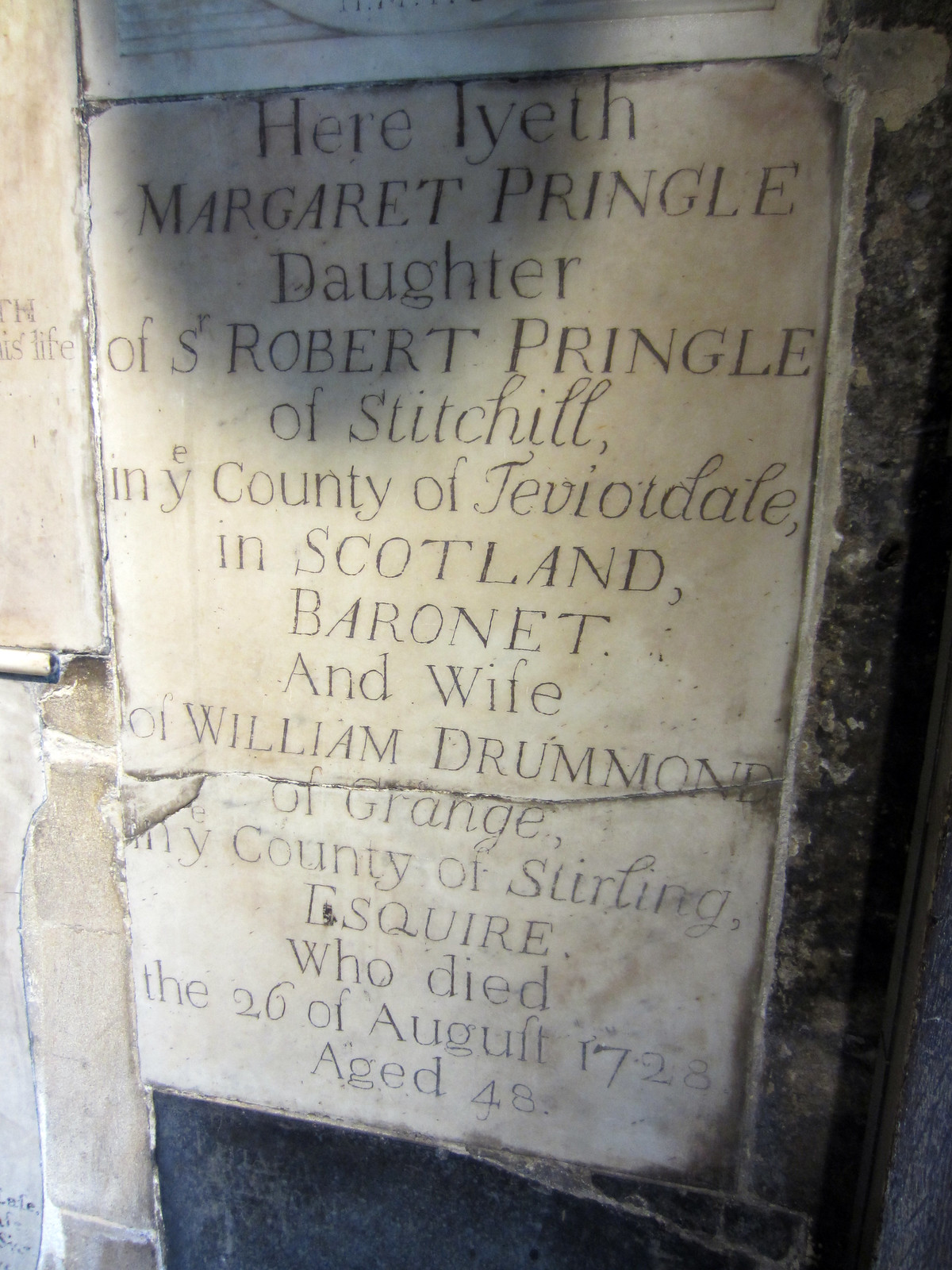This image depicts an ancient, weathered tombstone, light brown in color and appearing quite beaten up with visible cracks. The text is carved into the stone, which is surrounded by different types of stone: a similar stone to the left, a granite-like stone to the right, and a very dark stone underneath. The inscription, despite its age, reads:

"Here lieth Margaret Pringle, daughter of S. Robert Pringle of Stitchill in E. County of Teviotdale in Scotland, Baronet, and wife of William Drummond of Grange, my County of Stirling, Esquire, who died the 26th of August, 1728, aged 48."

Notably, the tombstone emphasizes Margaret Pringle’s lineage and marital connection, with prominence given to her father, Robert Pringle, over her husband, William Drummond.